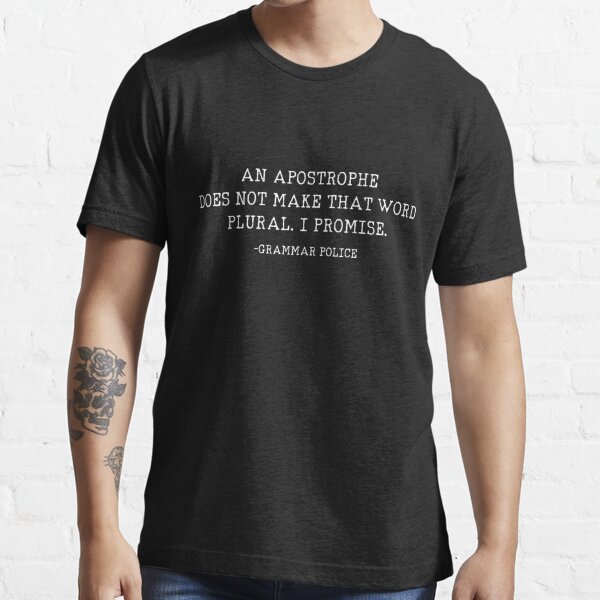The vertical rectangular image features a male model, depicted from just below the hips up to the neck, standing against a white-painted brick wall. He is of Caucasian descent and is dressed in jeans and a dark heather gray t-shirt with a crew neckline and short sleeves. The t-shirt bears a typewriter font message in white letters spanning four lines: “an apostrophe does not make that word plural. I promise. - Grammar Police.” On his right forearm, he has a detailed tattoo of a skull with a rose on top, entwined by a vine passing through the skull's eye sockets. The model’s face is not visible, as the image is cropped just below his chin, emphasizing the text on his shirt and his distinctive tattoo.